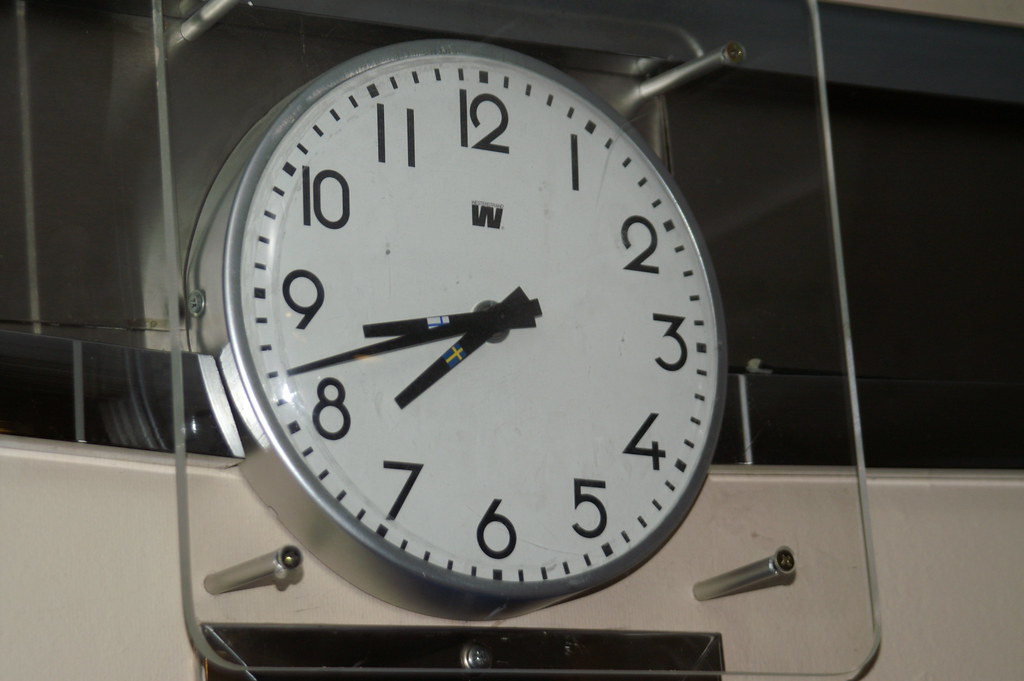This is a landscape-oriented photograph of an analogue clock, taken from a slight side angle, so the clock face is facing slightly to the right. The clock is encased in a transparent glass cover that is nailed in place with four screws, preventing direct contact. The clock features a silver-colored rim and a white face with large black numbers ranging from 1 to 12. The hands, which display the current time as approximately quarter to eight (with the small hand between 7 and 8, and the big hand between 8 and 9), are black and adorned with the flags of Sweden and Finland. The clock also features a 'W' logo at the top of the face. The entire setup is against a background that is a combination of dark grey, black, and cream-white colors.